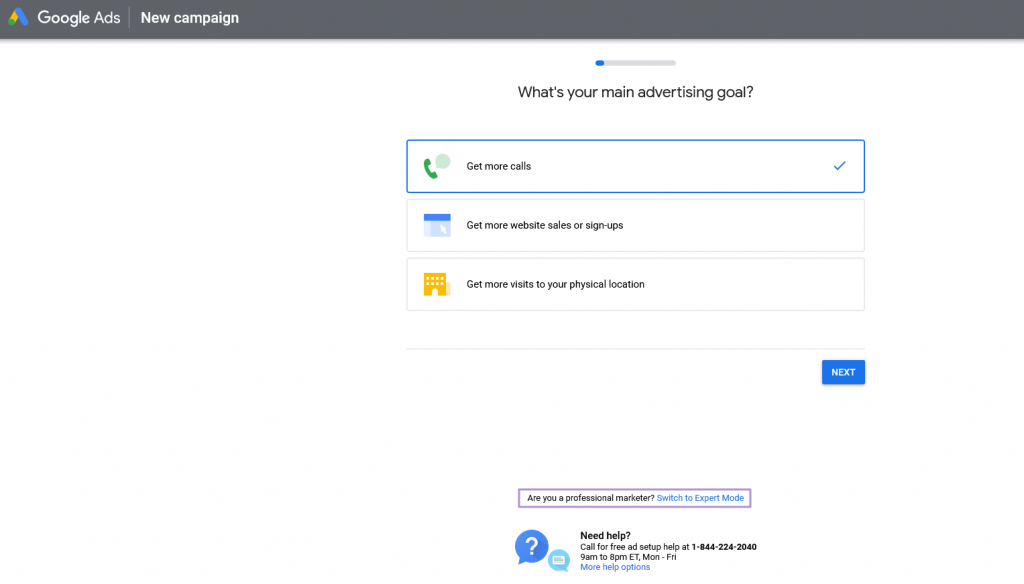The image depicts a Google Ads interface on a website. In the top left corner, the text "Google Ads" is displayed. To the right of this, "New Campaign" is written on a gray background.

Below, there is a progress bar – 90% of which is gray and 10% blue at the left end. Further down, the text "What's your main advertising goal?" appears, prompting the user to choose from three options:

1. "Get more calls" – Highlighted in blue with a green cell phone icon to the left.
2. "Get more website sales or signups".
3. "Get more visits to your physical location".

To the bottom right of these options is a blue square with "Next" written in white centered text.

Below the "Next" button, the text "Are you a professional marketer? Switch to expert mode" is displayed, with the latter part in light blue and the former in black. Beneath this, a blue circle with a question mark inside and a smaller, light blue (turquoise) circle bearing the text "Need Help?" followed by a phone number for assistance.

The entire interface is set against a clean, white background.